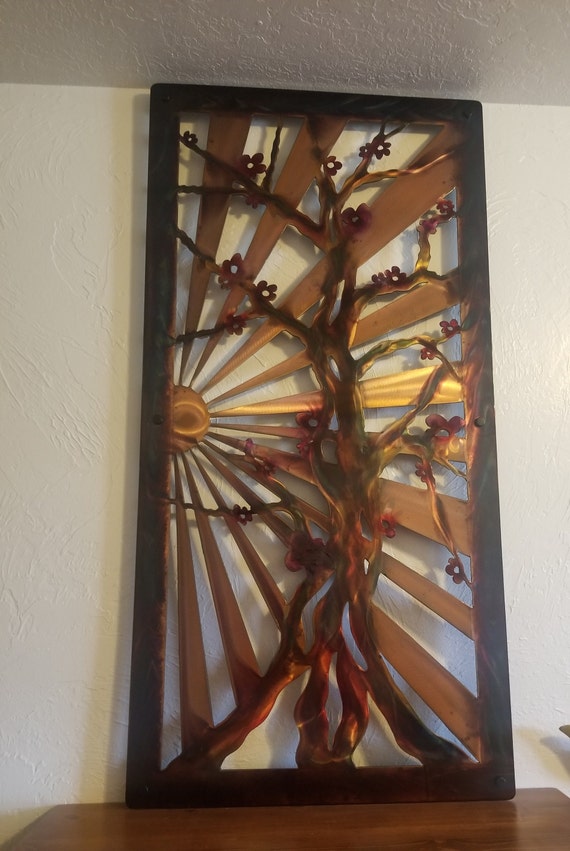This intricately carved artwork, housed within a rectangular cherry wood frame, evokes the serene beauty of Japan. The vertical frame, taller than it is wide, provides a sturdy anchor for the piece. In the background, a bronzed sun radiates beams of light from the left side, reminiscent of the old Rising Sun flag but rendered in warm bronze hues. These beams expand outward, symbolizing the sun's light reaching every corner of the world. Rising from the base are what appear to be cherry blossom trees, their twisted branches growing upwards into the sun's nurturing glow. This stunning piece sits elegantly on a table, its impressive height nearly touching the ceiling, inviting viewers to bask in its intricate details and tranquil aura.